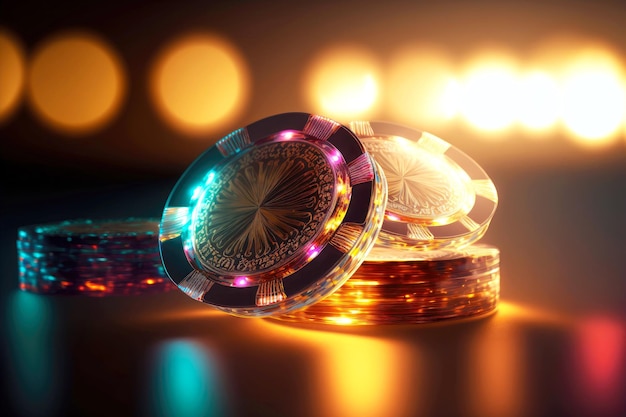The image depicts a close-up, possibly digitally-created or heavily edited photograph, of intricate, translucent poker chips that appear almost iridescent and ornamental. The central poker chip, prominently featuring a detailed, flower-like embossing, lies at an angle on top of two neat stacks of similar chips. These stacks and scattered chips exhibit alternating black and gold borders, with additional gold filigree enhancing their allure. They emit captivating LED-like lights, incorporating blue, purple, pink, and green hues that reflect and blend, resulting in a mesmerizing visual effect. The background is a dark, out-of-focus expanse dotted with blurred lights in white, red, blue, pink, orange, and yellow, creating a bokeh effect that resembles lens flares and adds depth to the scene. The surface on which the chips rest is reflective, amplifying the glow and further contributing to the photograph’s rich and elaborate aesthetic.